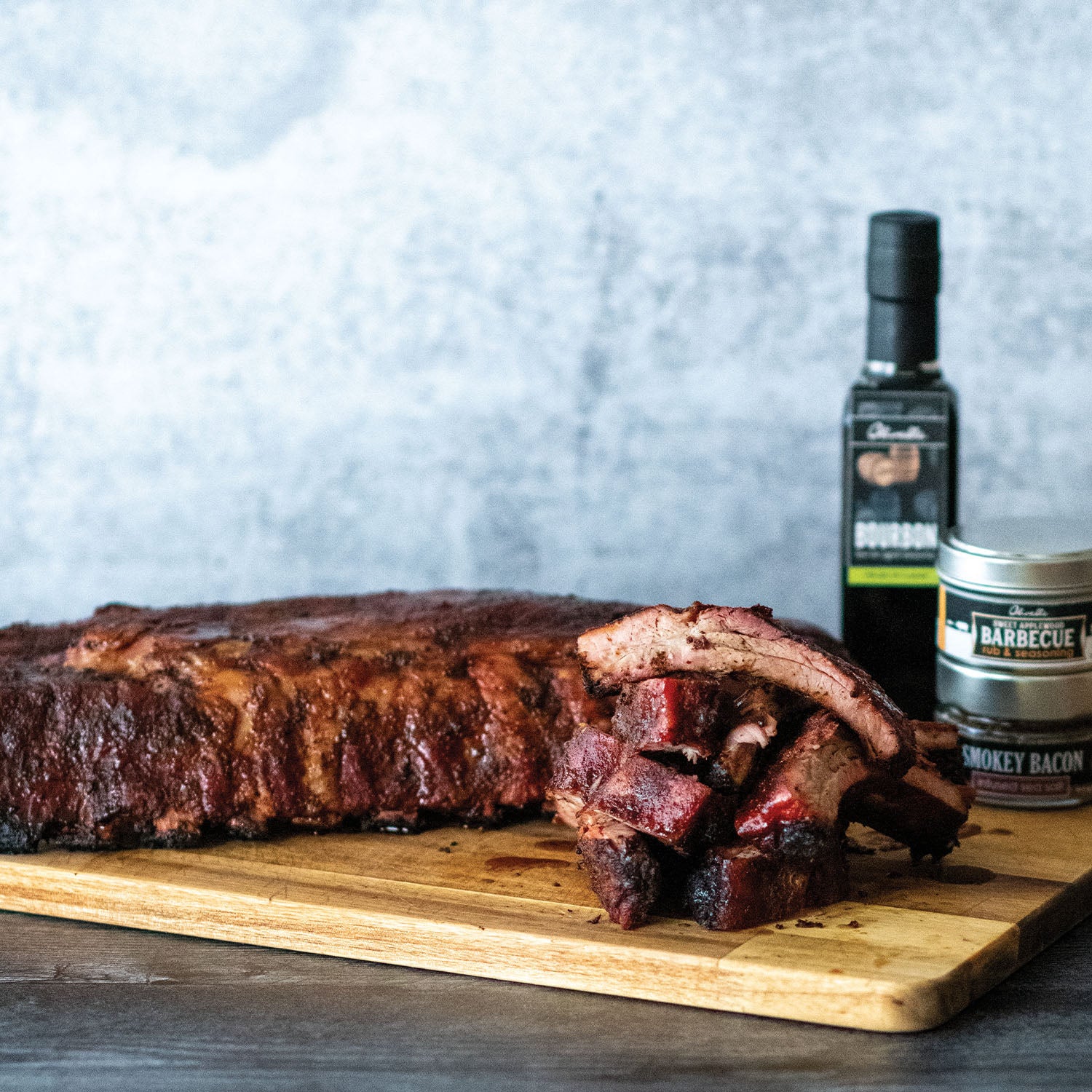The image showcases a perfectly cooked rack of barbecue spare ribs, deliciously browned and glistening with barbecue sauce. The ribs are artfully arranged on a thick brown cutting board, with some ribs already cut into individual pieces, displaying their juicy interiors. The cutting board rests on what appears to be a wooden table, though the lighting makes the exact material difficult to discern. In the background, there's a can labeled "barbecue" alongside a bottle whose label partially reads "bourbon.” The scene is complemented by jars of spices, including one labeled "smoky bacon." The overall presentation against a simple white backdrop emphasizes the succulent appearance of the ribs, making them the star of this mouthwatering display.